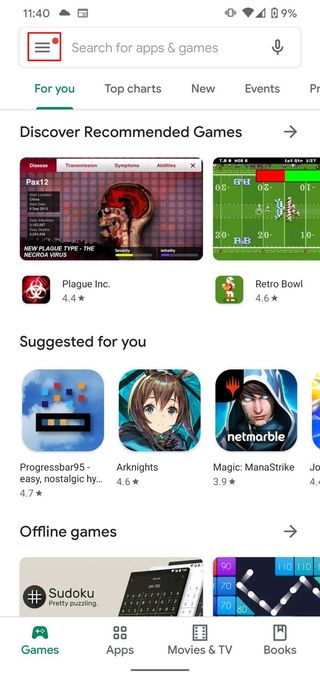This detailed and cleaned-up caption provides a comprehensive description of a screenshot from the Google Play Store captured on a mobile device:

The screenshot depicts the Google Play Store interface on a mobile device. In the top-left corner, a gray text displays the current time as "11:40." Next to this, three black lines represent a dropdown menu. Towards the top-right corner, a bold red circle, further emphasized by a squared red border, highlights an important element within the interface. This circle is situated within a light gray search query field that reads "Search for apps & games" with a medium gray microphone icon to its right, indicating the option for voice search.

Below the search bar, several menu options are presented. The first option, "For You," is highlighted in a bold teal color with an underline, indicating it is currently selected. Subsequent options include "Top Charts," "New Events," and a partially visible option starting with "P," all rendered in gray. 

A light gray horizontal line separates these menu options from the main content. On the left side, in black text, it states "Discover recommended games," accompanied by a medium gray arrow pointing to the right. 

The first game recommendation features a screenshot of a human skull and brain with the title "PAX 12" displayed in white text on the left side. Below this image, the game title "Plague Inc." is displayed with a rating of 4.4 stars, printed in gray text. Adjacent to this, another recommended game titled "Retro Bowl" is shown with a screenshot of a baseball field, boasting a rating of 4.6 stars, also shown in gray text.

Additionally, there is a menu element below the main header area, which has a highlighted option in red while the remaining options are in white with red text, suggesting a selectable list for navigation.